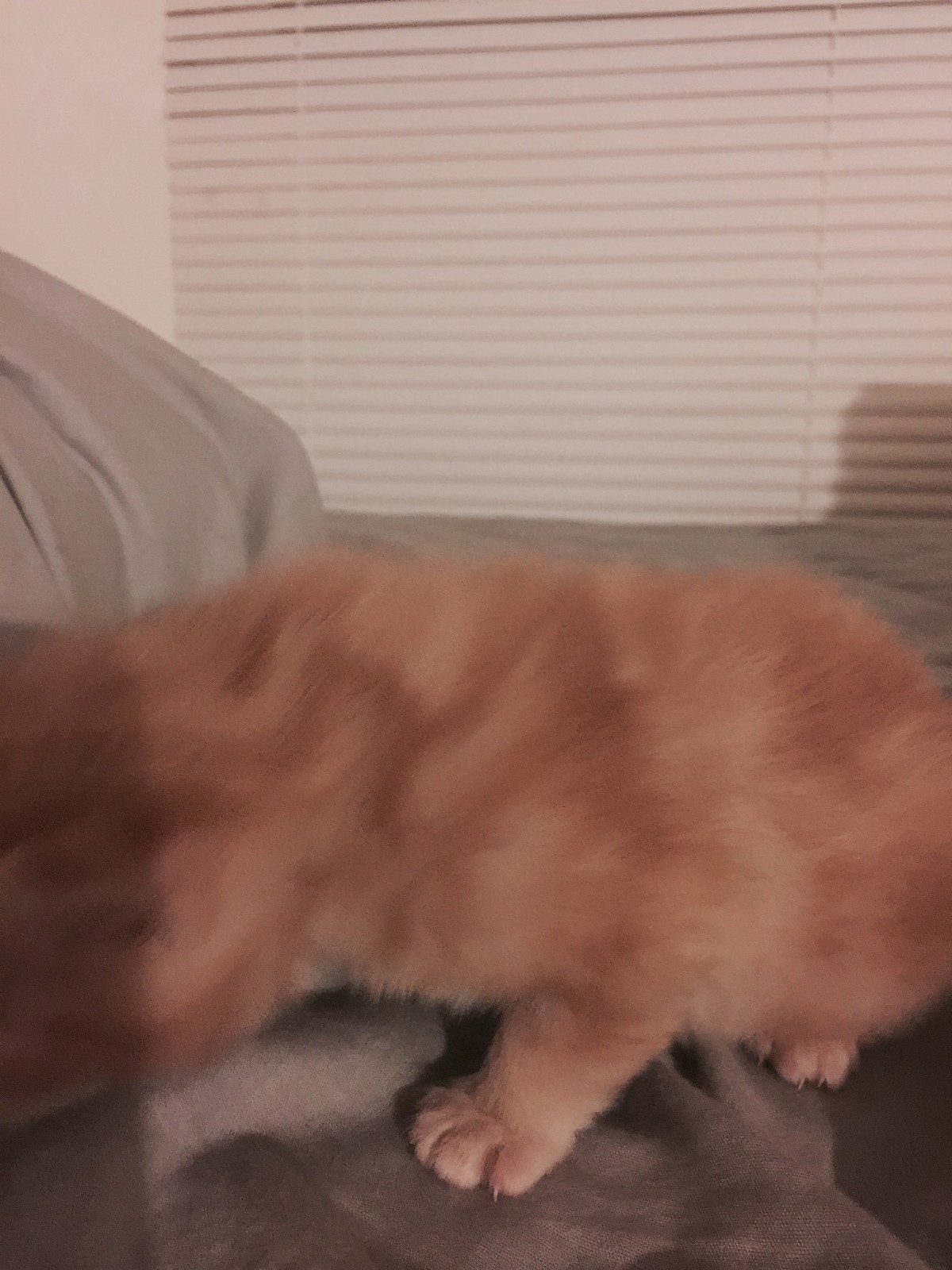The photograph captures a close-up view of an orange cat, predominantly showcasing its body, part of its head, and a couple of its paws. The feline appears to be standing on a plush gray comforter or blanket. The background features white blinds covering a window, with a slice of a white wall visible in the top left corner. A shadow is noticeable on the bottom right corner of the blinds. Despite the image being somewhat blurry and not of the highest quality, it distinctly highlights the cat as the main subject, positioned with its head facing down towards the gray blanket.